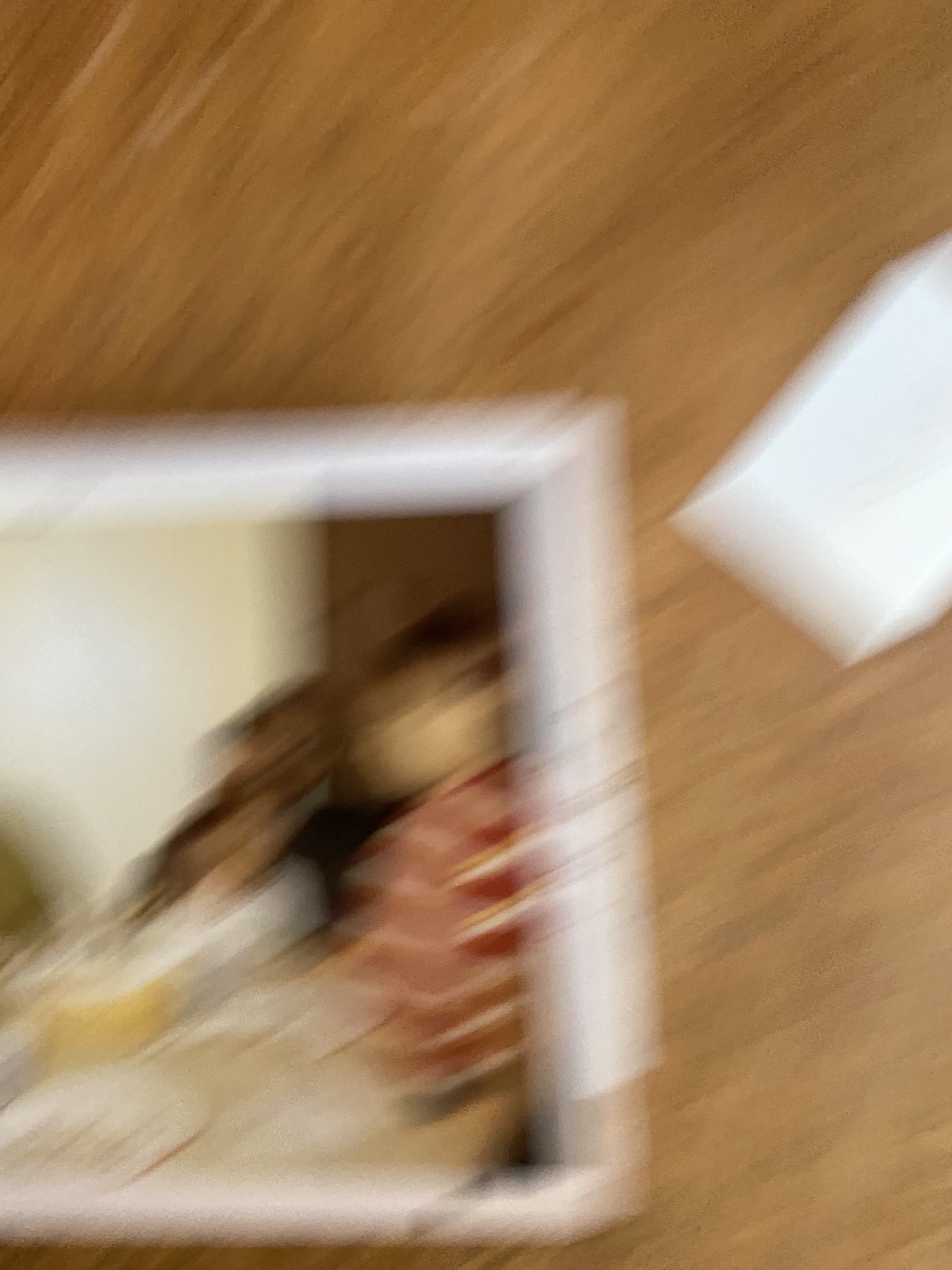This extremely blurry photograph captures what appears to be an image of a Polaroid or framed picture sitting on a medium-tone brown wooden table. The framed photo, located in the bottom left corner of the picture, is small—approximately 3x5 inches—and surrounded by a very thin white frame. The picture within the frame is difficult to discern due to the blur, but it seems to feature children or people sitting at a table, which has plates and pots on it. A notable detail includes a young person on the right side of the photo wearing a red and white striped shirt, with the blur causing the stripes to extend beyond the frame. Additionally, a white rectangular object is visible in the top right corner of the image, further adding to the complexity and indistinct quality of the scene.